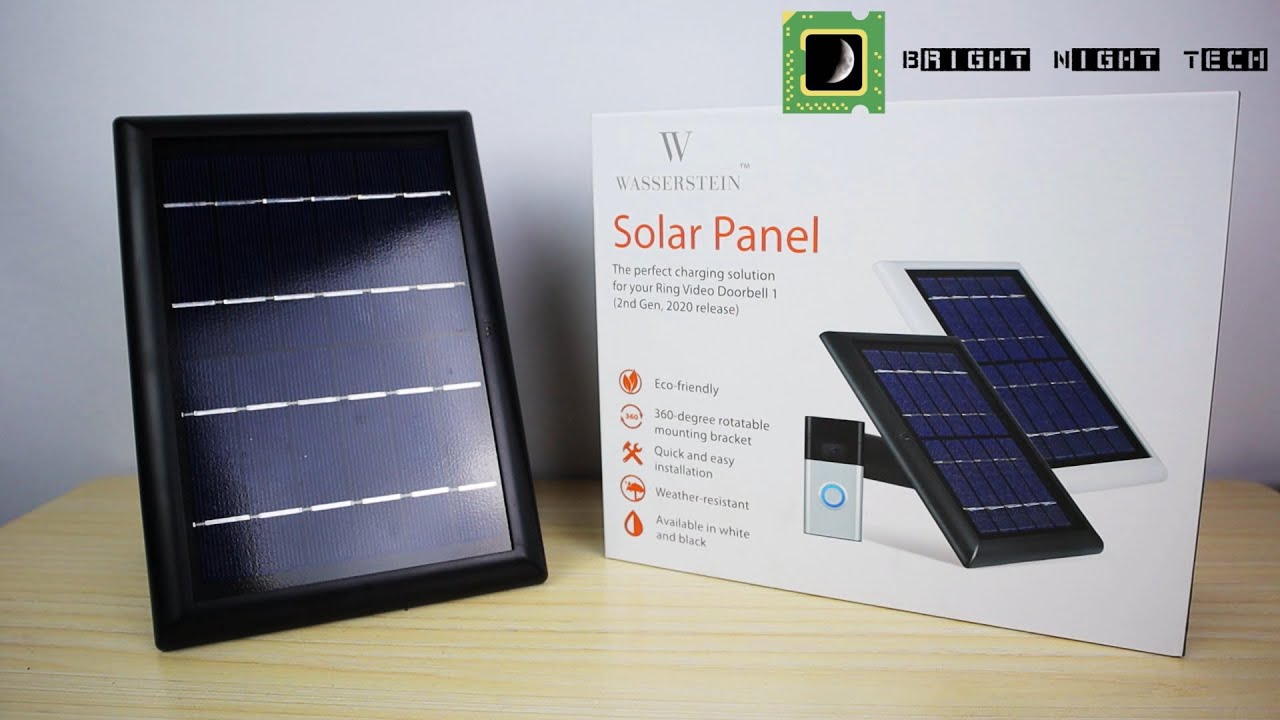The image showcases a product from Bright Night Tech, displayed on a light tan wooden table against a white wall. On the left side of the image is a black-framed Wasserstein solar panel with dark blue sections divided by white lines. To the right, there is a white box featuring two solar panels, one with a black frame and one with a white frame. The box includes text and icons detailing the product features: top left, it has "Wasserstein" accompanied by a letter "W" logo. Key features highlighted in orange or yellow include "the perfect charging solution for your Ring Doorbell 1, Second Generation 2020 release," "eco-friendly" with a leaf emoji, "360-degree rotatable mounting bracket," "quick and easy installation" with tool icons, "weather-resistant" with an umbrella and raindrop, and "available in black and white." Additionally, the top right of the box features the Bright Knight Tech logo, which resembles a green computer chip with a crescent moon and yellow-bordered stencil font.